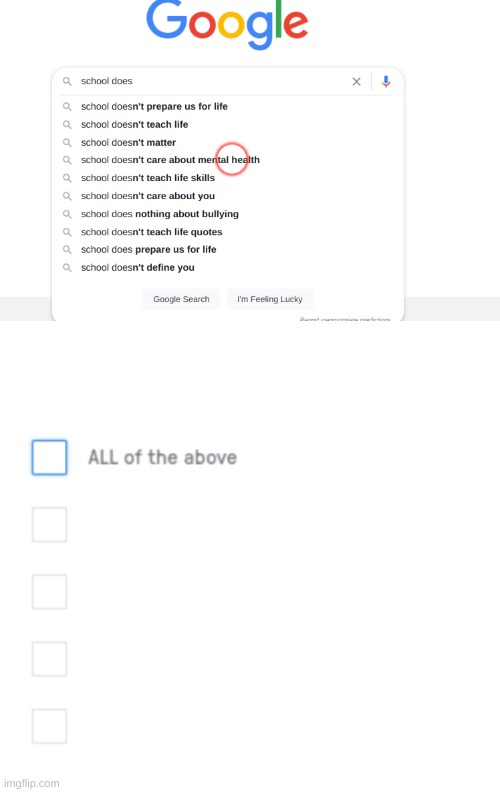The image displays a Google search page with a query in the search bar that reads "school doesn't." Below the search bar, a dropdown list of autocomplete suggestions is visible, offering various phrases including:

- "school doesn't prepare us for life"
- "school doesn't teach life"
- "school doesn't matter"
- "school doesn't care about mental health" (with a red circle marking parts of the words "mental" and "health")

Following this, more suggestions are visible, namely:
- "school doesn't teach life skills"
- "school doesn't care about you"
- "school does nothing about bullying"
- "school doesn't teach life quotes"
- "school does prepare us for life"
- "school doesn't define you"

Below these suggestions, there are the standard Google search buttons: "Google Search" and "I'm Feeling Lucky," both in gray. Beneath these buttons, five square gray boxes are present, with the top one highlighted in blue and labeled "all of the above," while the remaining four are empty and grayed out.

At the very bottom left-hand corner of the image, the watermark "imgflip.com" is visible, indicating the source of the image.